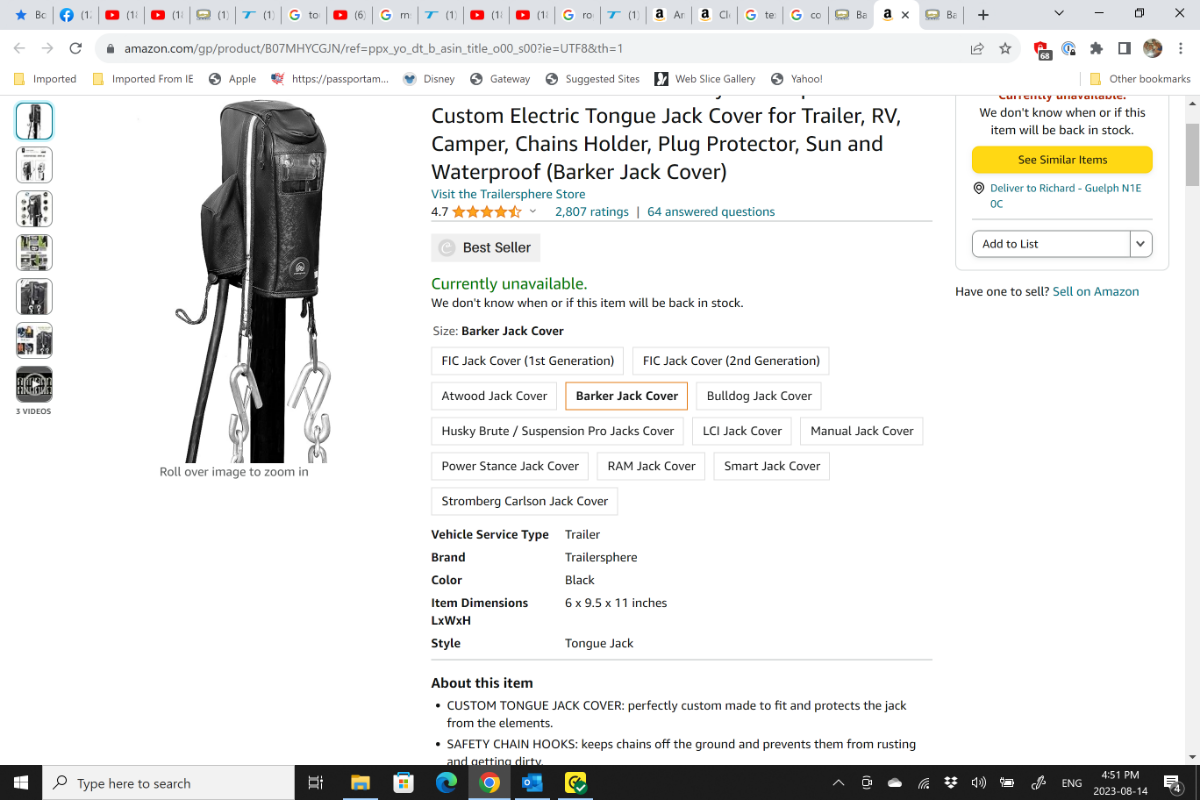A vibrant, full-color screenshot captures the entirety of a computer screen, where approximately 25 browser tabs are open. The active tab, second from the end, is displaying a product page on Amazon.com. The featured product is a custom electric tongue jack cover designed for trailers, RVs, and campers, equipped to hold chains, protect plugs, and shield against sun and water damage.

The product boasts an impressive 4.7-star rating based on 2,807 reviews, with 64 answered questions and a 'Bestseller' label. Despite its popularity, the item is currently marked as unavailable, indicated by a green notification stating, "We don't know when or if this item will be back in stock," and thus the 'Add to Cart' button is disabled.

The product page also offers three video demonstrations and a series of additional images that potential buyers can scroll through. To the right of the main display, there is an option to view similar items, providing alternatives given the unavailability of this specific product.